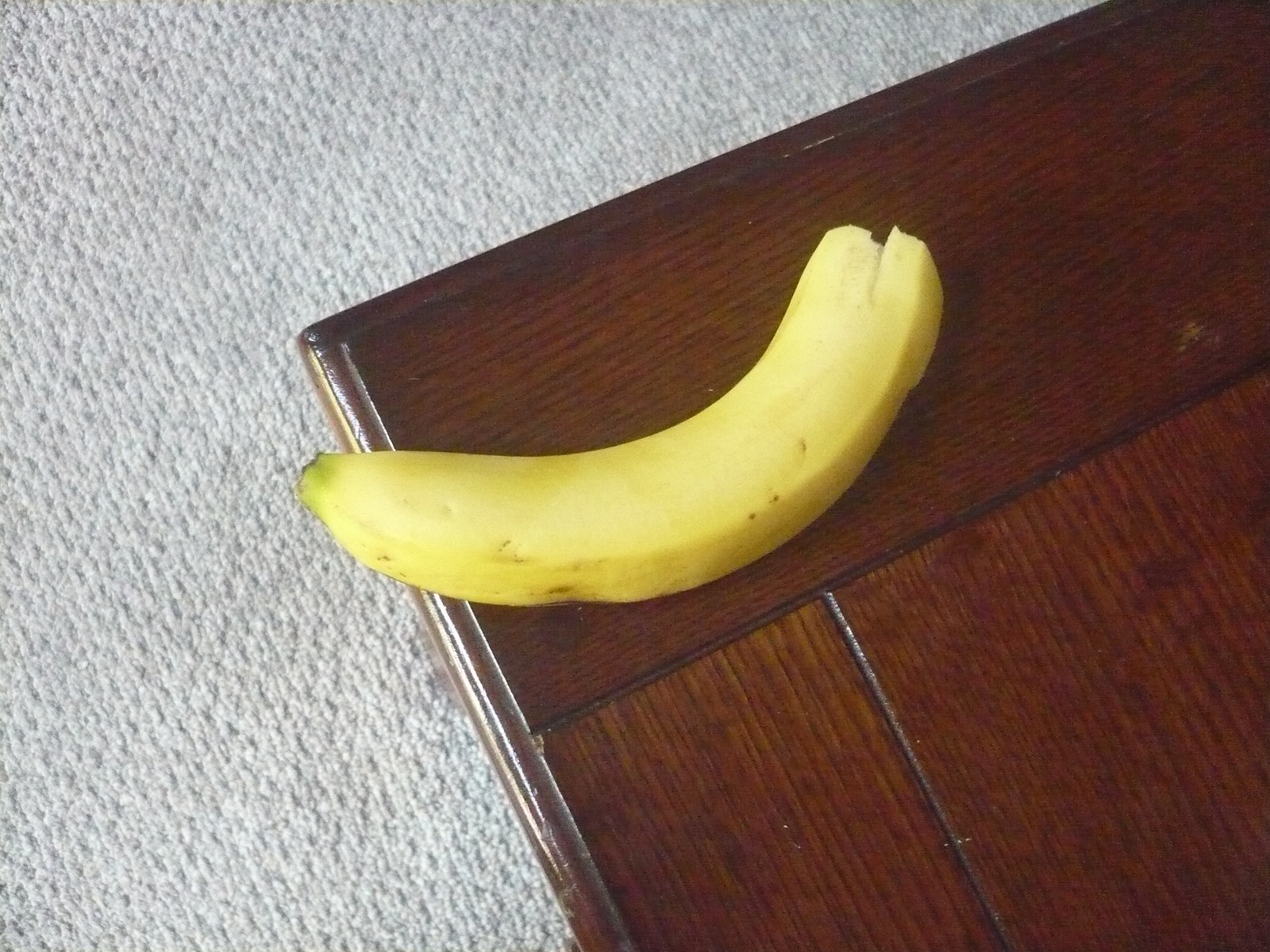This indoor photograph captures a detailed scene within a home's cozy setting. Central to the image, a dark wooden coffee table stands on a neutral-toned carpet, which boasts a creamy white hue interspersed with hints of brown. The coffee table, positioned on the left side of the frame, shows signs of wear, with visible scrapes and scratches marring its otherwise rich surface.

Prominently, a partially peeled yellow banana rests on the top left corner of the table, its end dangling slightly over the edge. The banana, though mostly fresh, exhibits a few brown spots indicative of ripening. The warm, inviting background highlights the contrast between the smooth carpet and the roughened wood of the coffee table. An intimate glimpse into daily life, the photograph's understated elements—coffee table, banana, and carpet—collectively tell a quiet vignette of homely simplicity.